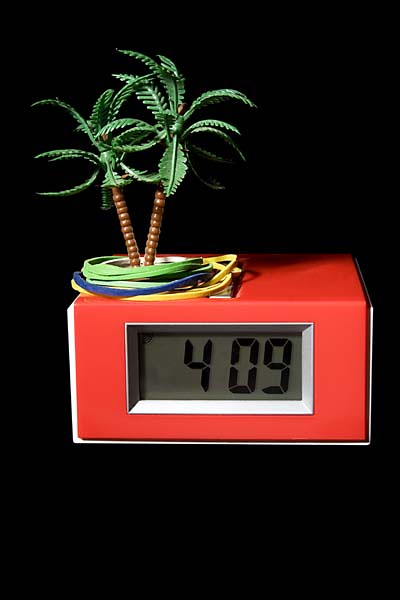The image shows a vintage-looking, bright red rectangular alarm clock with an LCD display that reads "4:09." The display features chunky black numbers on a dark background, surrounded by a white bezel. The clock evokes a design from the late 90s or early 2000s. Atop the clock, there are two small model palm trees with brown trunks, resembling Lego pieces, and green palm leaves. Around the base of these trees, variously-colored rubber bands in green, blue, and yellow are placed. The entire scene is set against a pitch-black background, highlighting the clock and its decorative elements.